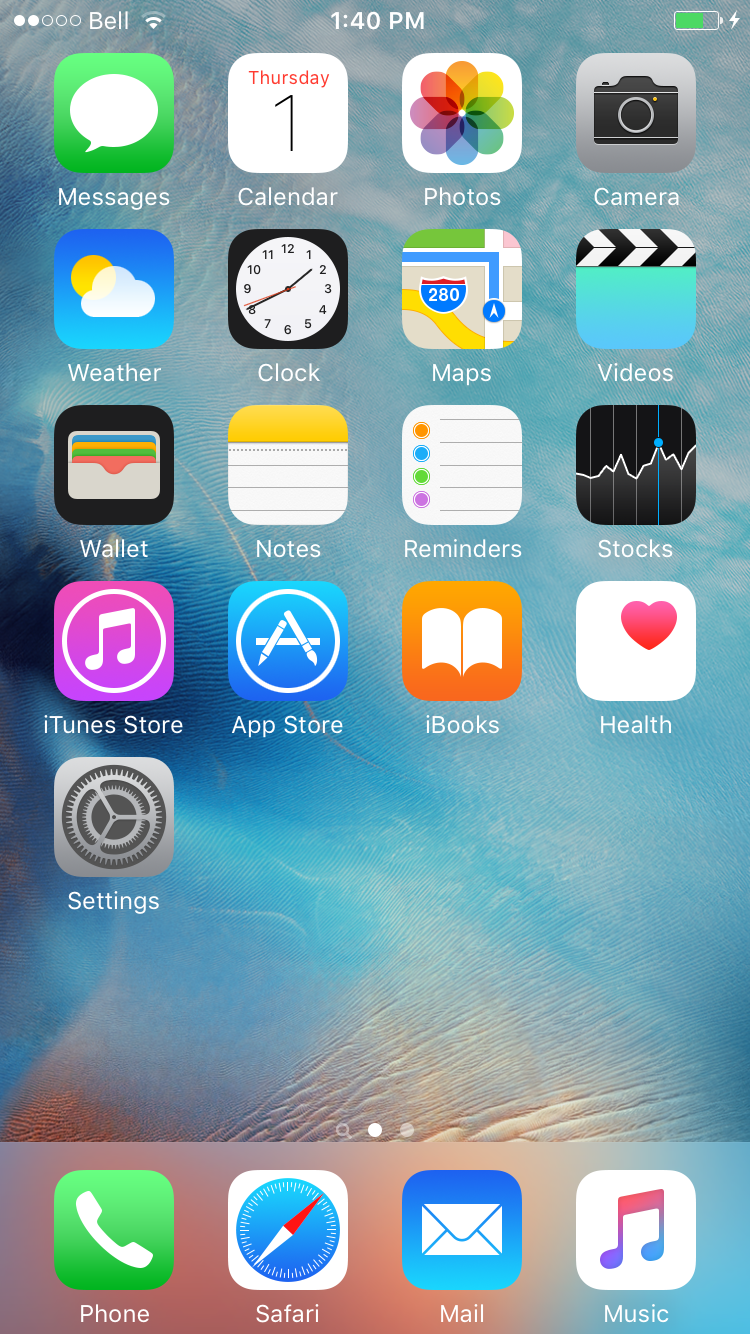Screenshot of a mobile phone home screen displayed at 1:40 PM, under the "Bell" Wi-Fi network, with roughly two-thirds battery life remaining. The background features a serene water texture with small ripples, blending from blue at the top to a pinkish hue near the bottom. The screen showcases four rows of four app icons each, along with a single icon at the bottom row. 

From the top left to right, the app icons are labeled as follows:
1. Messages
2. Calendar
3. Photos
4. Camera
5. Weather
6. Clock
7. Maps
8. Videos
9. Wallet
10. Notes
11. Reminders
12. Stocks
13. iTunes Store
14. App Store
15. Books
16. Health
17. Settings

Below this, situated on a fixed dock, are four additional app icons for quick access, labeled:
1. Phone
2. Safari
3. Mail
4. Music

The overall layout is symmetrical and consistent, with app names clearly visible beneath each icon. The background’s calming water texture contrasts smoothly with the vibrant app icons, creating an organized and aesthetically pleasing home screen.